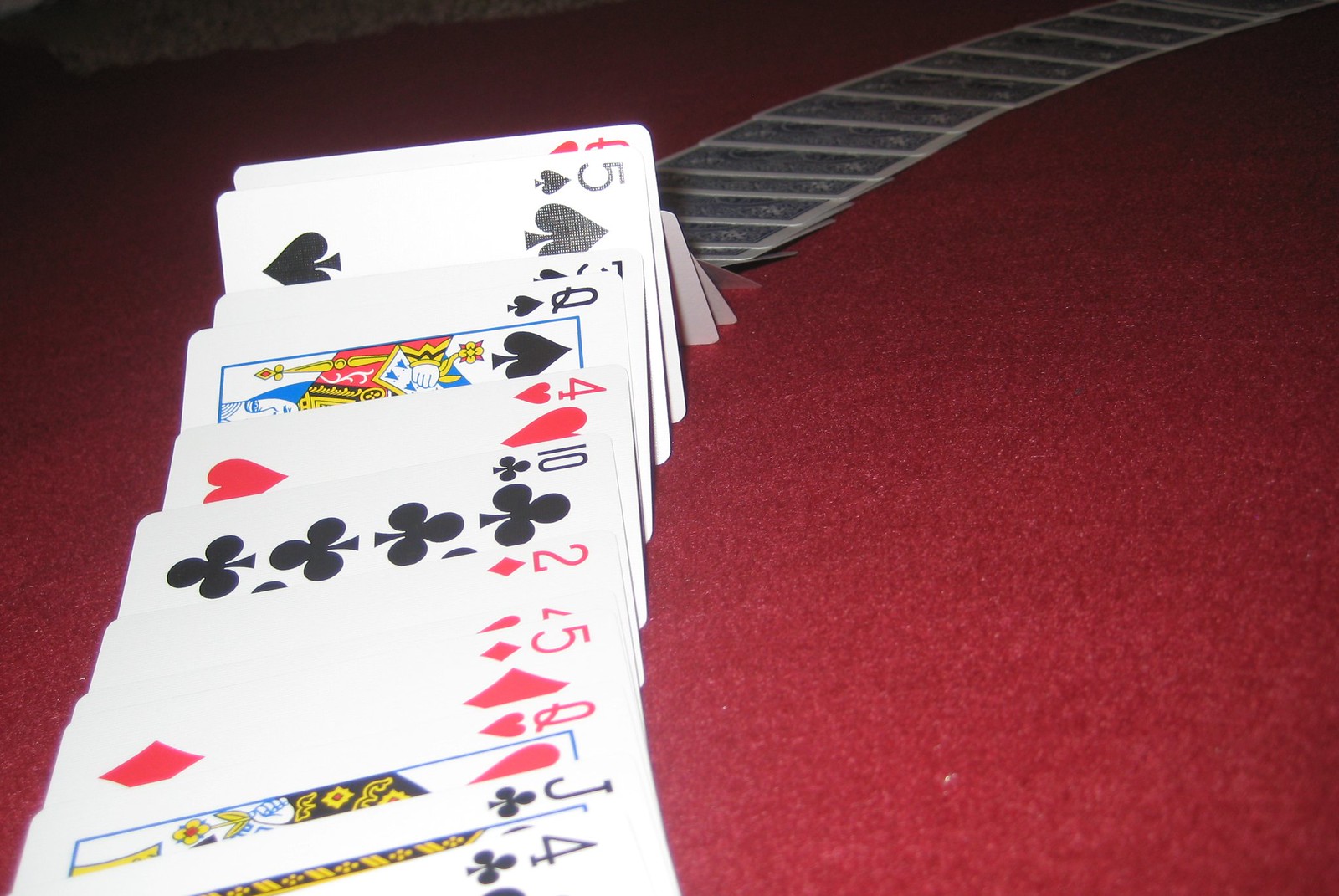A series of playing cards are laid out in a neat, sequential line on what appears to be a luxurious, red velvet surface, reminiscent of a casino table. The cards are initially laid face down, and someone, demonstrating exceptional dexterity and skill, has begun flipping them over in rapid succession from left to right. The image captures a moment mid-performance: approximately half of the cards lie face-up, while the other half remain face-down. The very first exposed card at the left edge of the frame is the Four of Clubs, and the sequence continues through a mix of different cards until the last visible flipped card, which is the Queen of Hearts. The rest of the cards awaiting revelation create an intriguing sense of anticipation. No person is visible in the image, yet the dynamic nature of the trick is palpable, highlighting the finesse required for such an act.